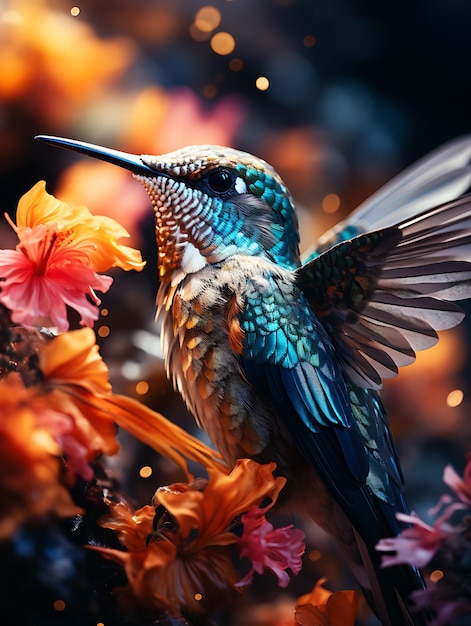This captivating close-up photograph showcases a stunning hummingbird in mid-flight, beautifully detailed and vividly colored. The hummingbird's bright blue, shiny feathers adorn its head, while its breast displays a striking orange hue complemented by gray feathers. The bird's long, slender black beak is poised towards a cluster of honeysuckle flowers, characterized by their pinkish and orange petals. The background is artistically blurred with hints of orange light, possibly from more flowers, creating a serene contrast that enhances the vivid focus on the hummingbird. The composition captures the dynamic elegance of the bird's wings, mid-beat, revealing the intricate mix of blue and gray on the feathers. The scene is a harmonious blend of vibrant colors and delicate details, meticulously capturing the ephemeral beauty of the hummingbird and its floral surroundings.